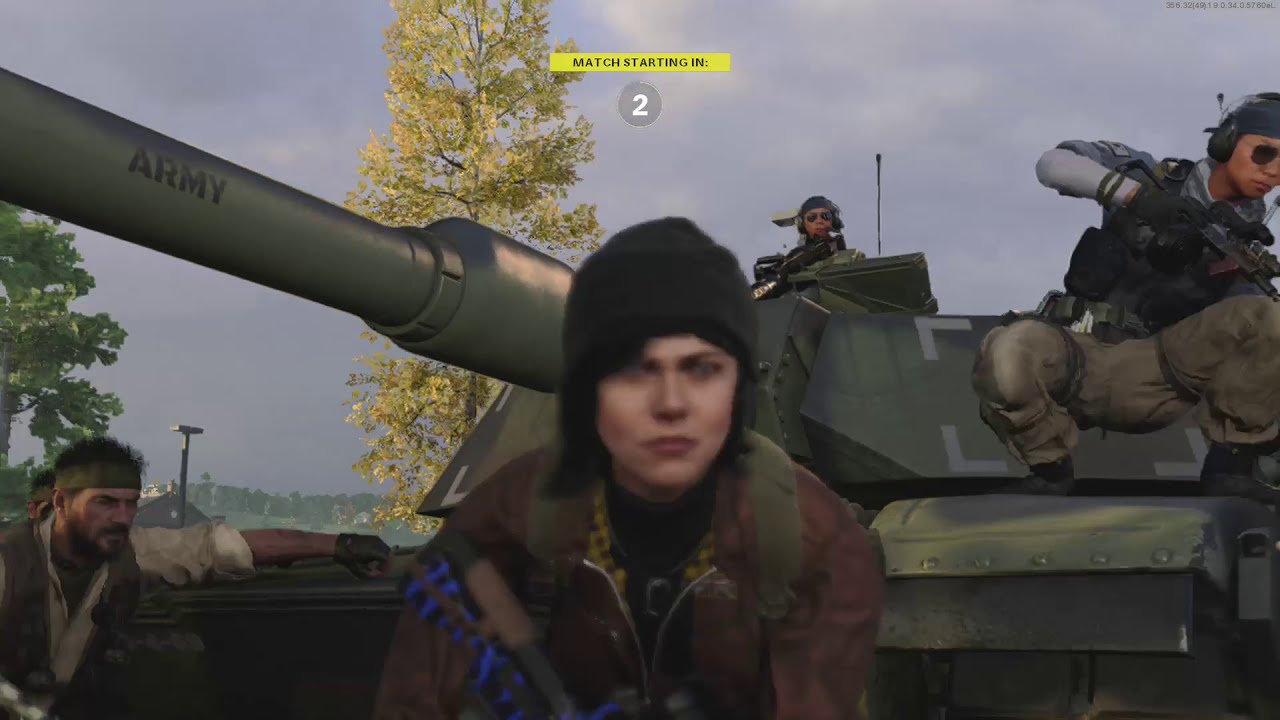This is a detailed, computer-generated image resembling a video game screenshot with the text "match starting in" displayed at the top in yellow, with a small "2" inside a gray circle at the forefront. The scene is set outdoors with various features.

Central to the image is a young Caucasian woman in her early 20s, sporting short black hair and a black knit skullcap. She is attired in a brown leather bombardier jacket with a yellow and black checkered shirt peeking out and a black turtleneck. A green backpack strap is visible over her right shoulder, and she holds a weapon angled downward. She looks directly at the camera with an intense expression, though the lower half of her body is cut off.

Behind her is a large, dark green army tank extending from the right side to slightly past the middle of the image. The tank barrel, labeled "army" in black letters, stretches diagonally over her shoulder. Atop the tank turret is a man wearing fatigues, a helmet, sunglasses, and a headset, possibly communicating through a microphone. To his right, protruding halfway off the image, is another soldier with dark sunglasses, a gray long-sleeve shirt, and black gloves.

On the left side of the tank stands a man with a full mustache and beard, dark hair, a green headband, and an open-collared white shirt with rolled-up sleeves and gloves, over which he has a vest. He leans slightly forward and faces the tank and woman. The background features a landscape with sloping mountains, buildings or hangars, and two distinct trees—a healthy one with green leaves on the left and another with yellowing leaves in the middle background.

The sky is a grayish-blue, adding to the intense atmosphere of the scene.